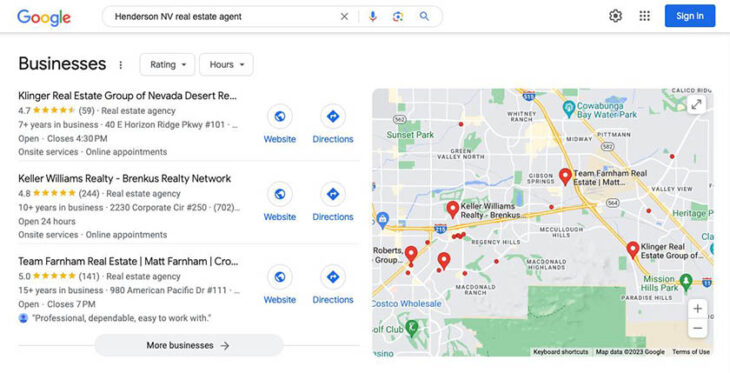Screenshot of Google Maps search results with the query "Henderson Envy Real Estate Agent." The top header is white with the Google logo on the left and a search bar to its right containing the query text. To the right of the search bar, there are a cog icon, a grid of nine dots, and a blue sign-in button.

Below the header, the search results are categorized under "Businesses" in bold black text, followed by three vertical dots and two drop-down menus labeled "Rating" and "Hours." The interface displays a city map in the Google Maps style on the bottom right, marked with several red pins indicating locations.

To the left of the map, three search results are listed:

1. **Klinger Real Estate Group of Nevada Desert**
   - **Rating**: 4.7 stars, based on 59 reviews
   - **Category**: Real estate agency
   - **Years in Business**: 7+ years
   - **Address**: 40 East Horizon Ridge Parkway, Number 101
   - **Hours**: Open, closes at 4:30 PM
   - **Services**: On-site services, online appointments
   - **Icons**: Website, Directions

2. **Keller Williams Realty, Brenkus Realty Network**
   - **Rating**: 4.8 stars, based on 244 reviews
   - **Category**: Real estate agency
   - **Years in Business**: 10+ years
   - **Address**: 2230 Corporate Circle, Number 250702
   - **Hours**: Open 24 hours
   - **Services**: On-site services, online appointments
   - **Icons**: Website, Directions

3. **Team Farnham Real Estate, Matt Farnham**
   - **Rating**: 5 stars, based on 141 reviews
   - **Category**: Real estate agency
   - **Years in Business**: 15+ years
   - **Address**: 980 American Pacific Drive, Number 111
   - **Hours**: Open, closes at 7:00 PM
   - **Icons**: Website, Directions
   - **Highlighted Review**: "Professional, dependable, easy to work with"